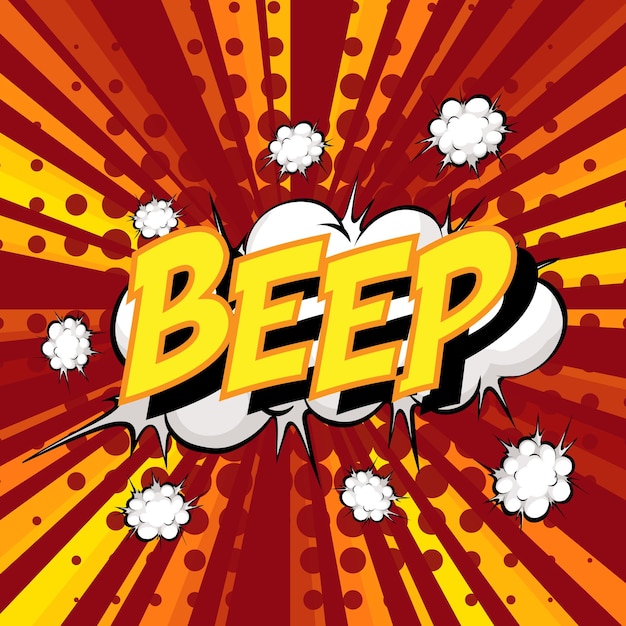This vibrant comic book-style illustration showcases the word "BEEP" prominently in the center, rendered in bold bright yellow letters with a golden border and a subtle black shadow. Surrounding the large central text is a dynamic arrangement of white clouds, featuring one large smoke cloud directly behind the letters and seven smaller smoke clouds sprouting from it. Emitting from the background are radiant rays and dots in a striking palette of crimson red, golden yellow, and orange, creating a sunburst effect that adds to the explosive, energetic feel of the image. The entire composition captures the dynamic, action-packed essence typical of comic book illustrations.